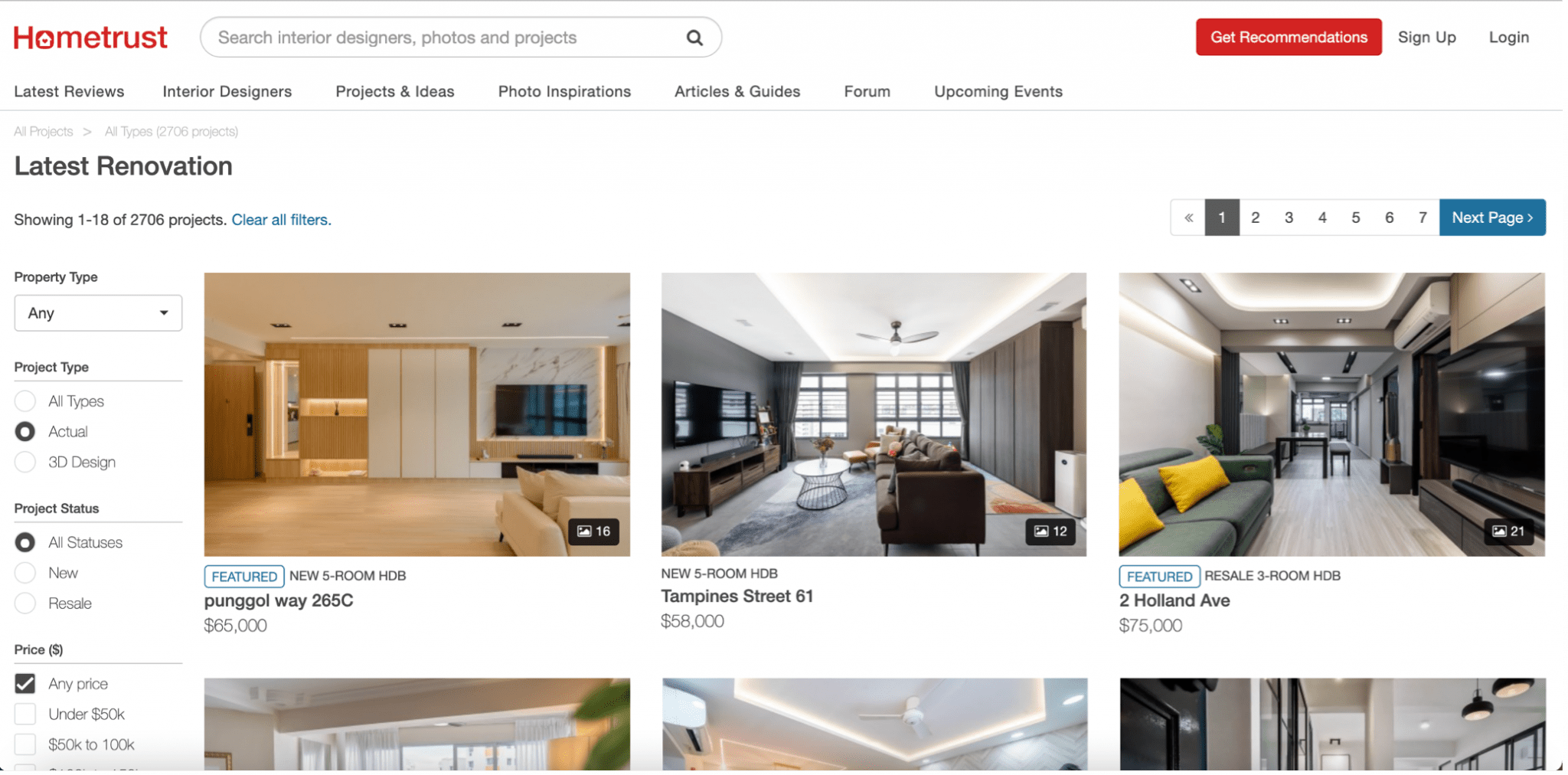This image is a screenshot of the HomeTrust website, a platform dedicated to providing inspiration and resources for home renovations and interior design. The interface features a pristine white background. Prominently displayed in the top left corner is the logo and site name, "HomeTrust," in striking red text. Centrally positioned at the top of the page is a search bar, allowing users to explore the website's extensive content. 

On the top right, a large red box with white text invites visitors to "Get Recommendations," facilitating personalized suggestions for home improvement. Adjacent to this call-to-action, in subtle gray text, are the "Sign Up" and "Log In" options, offering users access to personalized accounts.

Dominating the central portion of the page are multiple photographs showcasing recently completed home renovation projects. Each image is accompanied by detailed captions that include the address of the renovated property, a brief description of the specific room or area that was updated, and the cost of the renovation, which ranges between $58,000 and $75,000. These visuals serve as a rich source of ideas for potential renovations.

Additionally, the website provides links to various resources, such as interior designers, specific project ideas, and a wealth of articles and guides. These materials are designed to inspire and assist users in planning their renovations or in collaborating with professionals for their home improvement needs.